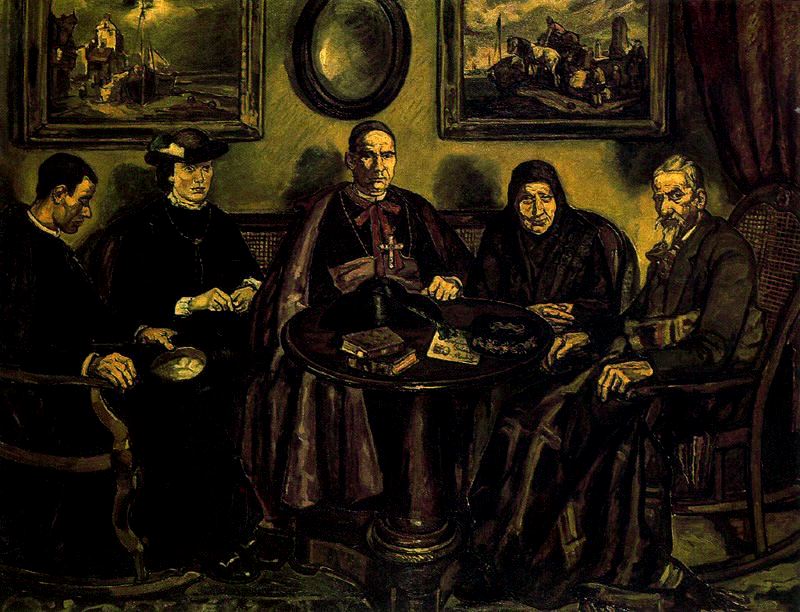This evocative and dark-toned painting depicts five somber individuals, centrally featuring a figure likely representing an archbishop or a pastor adorned with a large cross around their neck. They are gathered around a table adorned with books, suggesting a setting of religious or formal discourse. Flanking the central figure are two men and two women, all of whom display expressions of deep unhappiness or solemn contemplation. The backdrop features two wooden-framed paintings: one on the left showcasing a serene waterside scene with a house, and one on the right displaying a rider on horseback. A mirror is positioned at the top center of the background, adding to the layered and reflective nature of the scene. The painting is heavy with dark hues—primarily blacks, dark greens, browns, and touches of dark red and blue—emphasizing the weighty atmosphere and somber tone of the gathering. The overall style of the painting might suggest an allegorical critique or commentary on the influence and authority of the Catholic Church, potentially placing the religious figure in a central, unifying role amidst the surrounding figures.